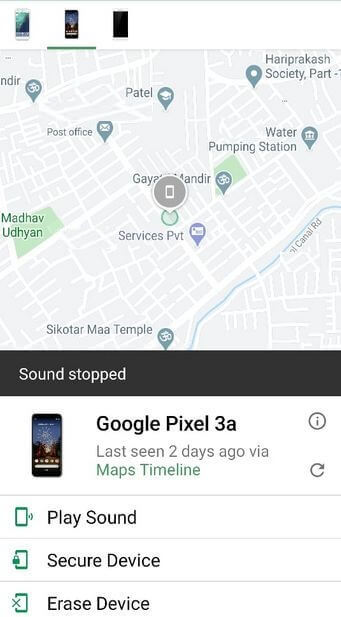The screenshot displays a web page showcasing an app with multiple sections and visual elements. Across the top, three phones are displayed: one with a blue and cyan background resembling water, another featuring a dark blue sky with black silhouettes beneath it, and a third phone that is entirely black.

Beneath this, a small rectangle reveals a street view map, showing several buildings labeled in dark gray, and streets marked with white rectangles. Multiple pins are located on the map, each representing different icons: a bike, an envelope, a cap, a dot, a museum, another bike, and a letter. Toward the center of these icons, there's a green circle encapsulating a phone and a large dark gray circle outlined in white. To the left, the text "Services PBT" appears in black.

Below this section, the display features a black bezel with the text "Sound Stopped" in white. Under this notification, an image of a Google Pixel phone is shown, encased in a black bezel. The screen displays a scenic image of trees in red and brown hues against a blue sky with stars. To the right of the phone, the text reads "Google Pixel 3A" alongside a gray information bubble.

Underneath this description, it notes "Last seen two days ago via Maps Timeline." Following this, three sections are displayed: the first shows a sound icon with the text "Play Sound," the second has a lock icon labeled "Secure Device," and the final section has an X icon labeled "Erase Device."